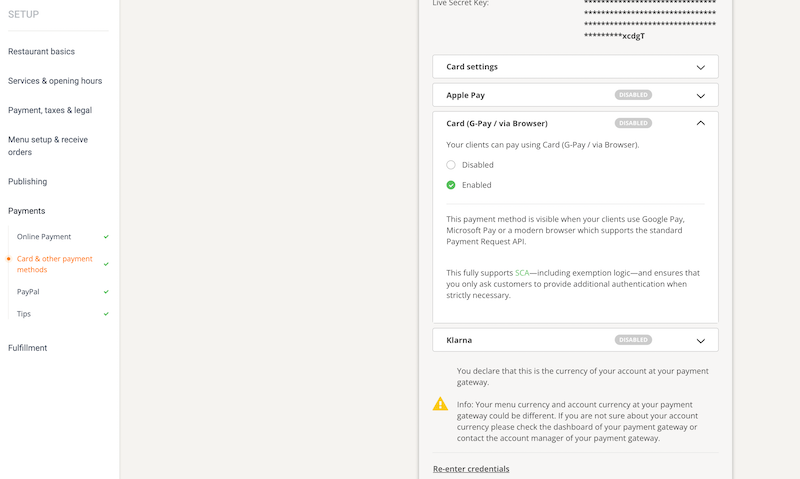Detailed Caption:
"The image depicts a section of a website dedicated to setting up various aspects of a restaurant business. The left sidebar features a comprehensive menu including options such as 'Setup,' 'Restaurant Basics,' 'Services and Opening Hours,' 'Payment,' 'Taxes and Legal,' 'Menu Setup and Receive Orders,' 'Publishing,' 'Payments,' and 'Fulfillment.' The current focus is on the 'Payment' section, and specifically within that, the subsection titled 'Card and Other Payment Methods.'

In the main content area on the right, users can configure payment options. The interface shows a list of selectable payment methods including Debit Card, Apple Pay, and GPay. GPay (Google Pay) is highlighted with the label 'Card (GPay/Via Browser)' indicating that this payment method has been enabled. Options to enable or disable this method are present, with 'Enable' currently active.

Below the selection, there is informative text explaining that this payment method becomes available to customers using Google Pay, Microsoft Pay, or any modern browser supporting the standard Payment Request API. This ensures full compatibility with contemporary digital payment systems. The setup is designed to allow restaurants to accept various forms of digital payments seamlessly."